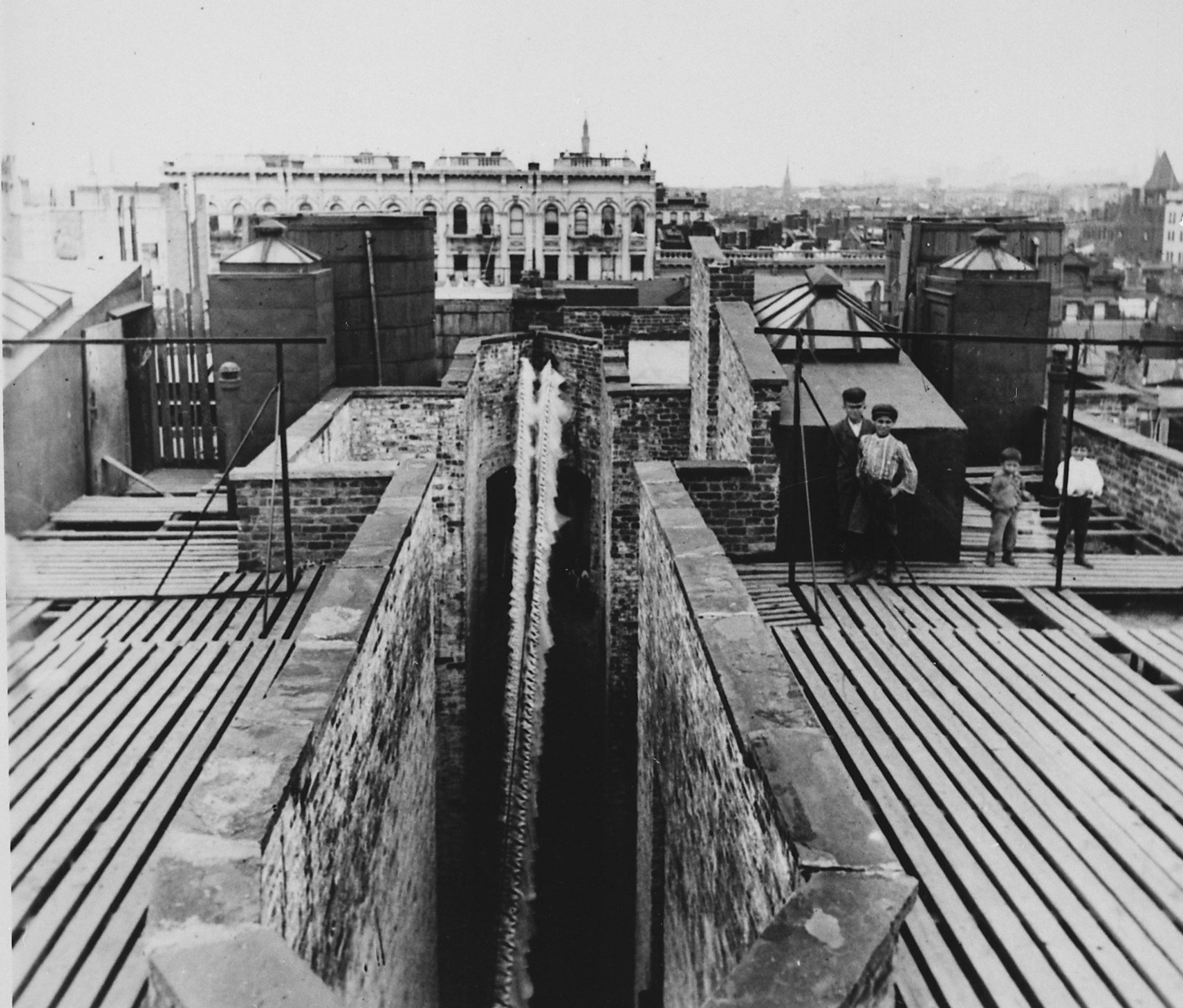In this horizontal, black and white photograph, likely taken many decades ago, we see the rooftop of perhaps one or two adjacent brick buildings. The central gap between the structures creates a sense of height and depth, with wooden planks laid across the rooftops. On the far right side, four boys stand on the roof, dressed in attire reminiscent of the 1920s, including long shirts and hats, suggesting their ages range from younger to older youths. A stream of water appears to be flowing from an indeterminate source on the roof, adding an element of mystery to the scene. The background reveals a cityscape consisting of more old buildings under a gray, overcast sky, emphasizing the historical context of the photograph.